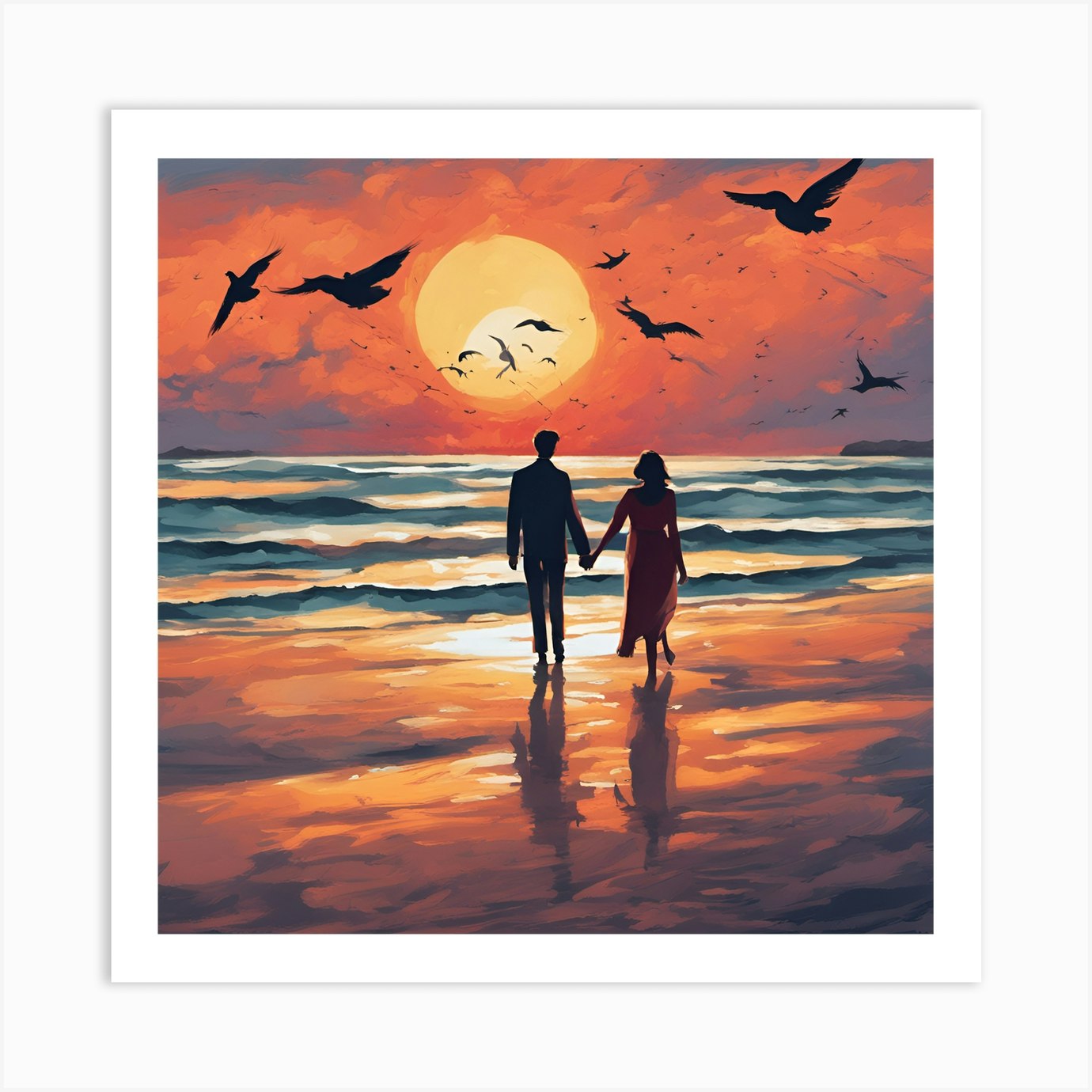This captivating painting, presented within a perfectly square frame with a white border, depicts a serene beach scene at sunset, designed to evoke nostalgic Polaroid imagery. Within the inner white border, the setting sun bathes the sky in shades of bright yellow, dull yellow, and rich orange hues, casting an enchanting glow over the tranquil ocean waves gently rippling towards the shore. Centered in the composition, a couple walks hand-in-hand towards the water, their backs facing the viewer. The man, likely dressed in a suit and pants, is positioned on the left, while the woman, donning a slightly sheer red dress that subtly reveals the outline of her lower legs, stands to his right. The duo's mutual stride, with the man's right leg forward and the woman’s right leg slightly raised, adds a dynamic element to their promenade. Shadows of the couple stretch out behind them on the wet sand, a testament to the setting sun's low angle. Above, numerous black silhouettes of seagulls, pelicans, and other birds punctuate the sky, enhancing the painting's sense of depth and liveliness as they vary in size, suggesting proximity to the viewer. This detailed portrayal captures an intimate and picturesque moment, blending natural beauty with human connection.